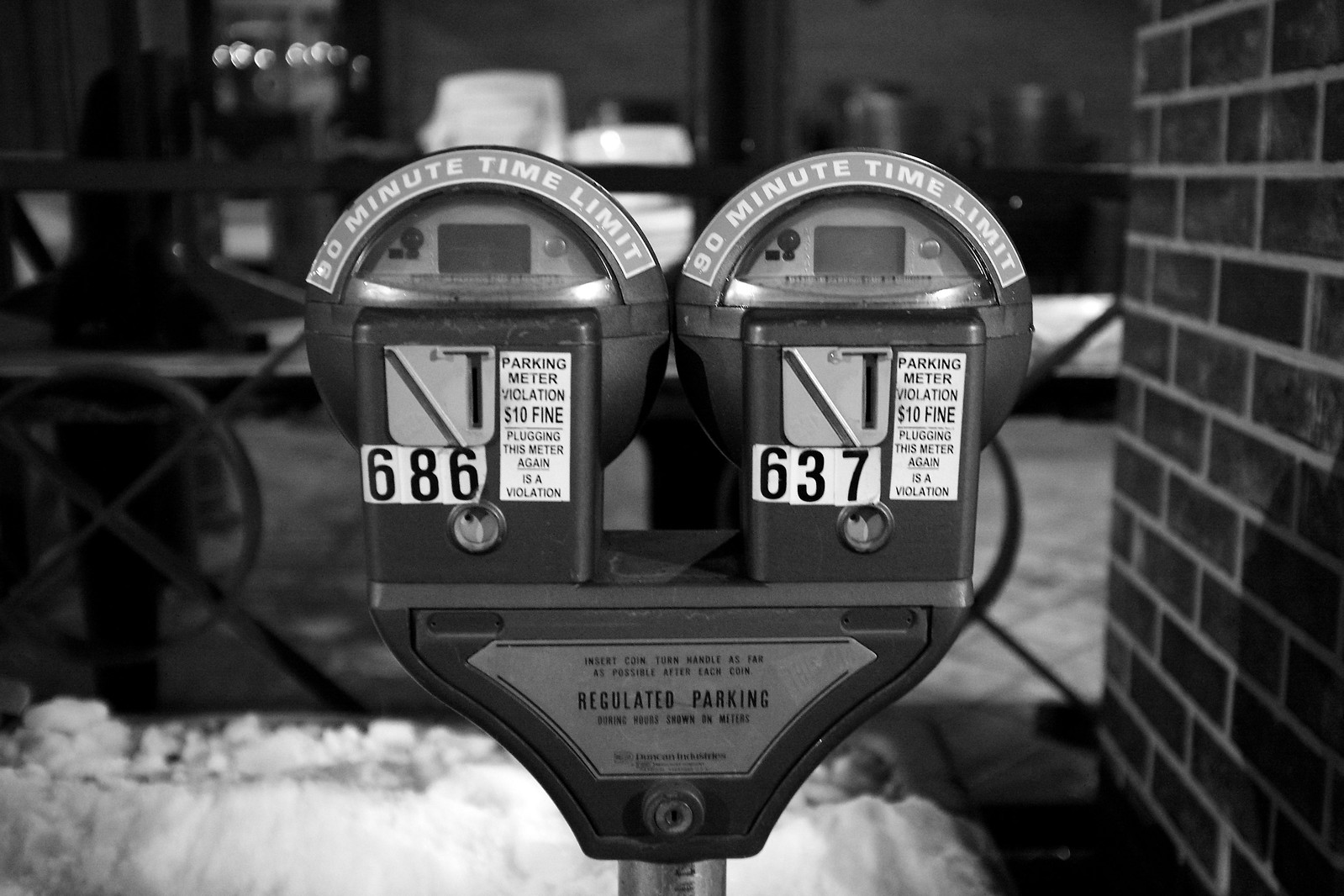This black and white photograph depicts a dual parking meter in a street scene, likely from the winter season given the snow visible on the ground. Positioned on a silver metal pole, bolted to the ground, the two meters share a single base. Each meter features a curved top labeled with a "90 minute time limit." The left meter is marked with the number 686 while the right one reads 637; both display slightly peeling stickers. Below the coin slots, there are white signs stating "Parking meter violation $10 fine. Plugging this meter again is a violation." The base of the meters is inscribed with "regulated parking." In the background, a grey brick wall is discernible, with blurry buildings further off in the distance, enhancing the vintage charm of this likely mid-20th-century image.